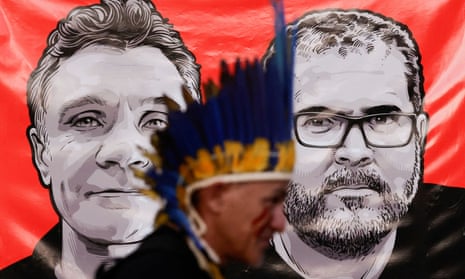This photograph captures a dynamic scene featuring a Native American man in the foreground, adorned with a traditional headdress that boasts vibrant yellow and bright blue feathers. He has red paint lines running from under his eyes down his cheeks. The man appears slightly out of focus as he gazes to the right. Behind him, the background is sharper, revealing a red tapestry decorated with detailed drawings of two middle-aged men's faces. The man on the left has short white hair and a clean-shaven, smiling expression, while the man on the right sports short, darker hair, a trimmed beard, and black-rimmed prescription glasses. Both men in the drawing seem to be of European descent and are depicted in black and white against the red backdrop. The overall composition highlights the contrast between the vivid presence of the Native American man and the striking, yet static, artistic representations behind him.